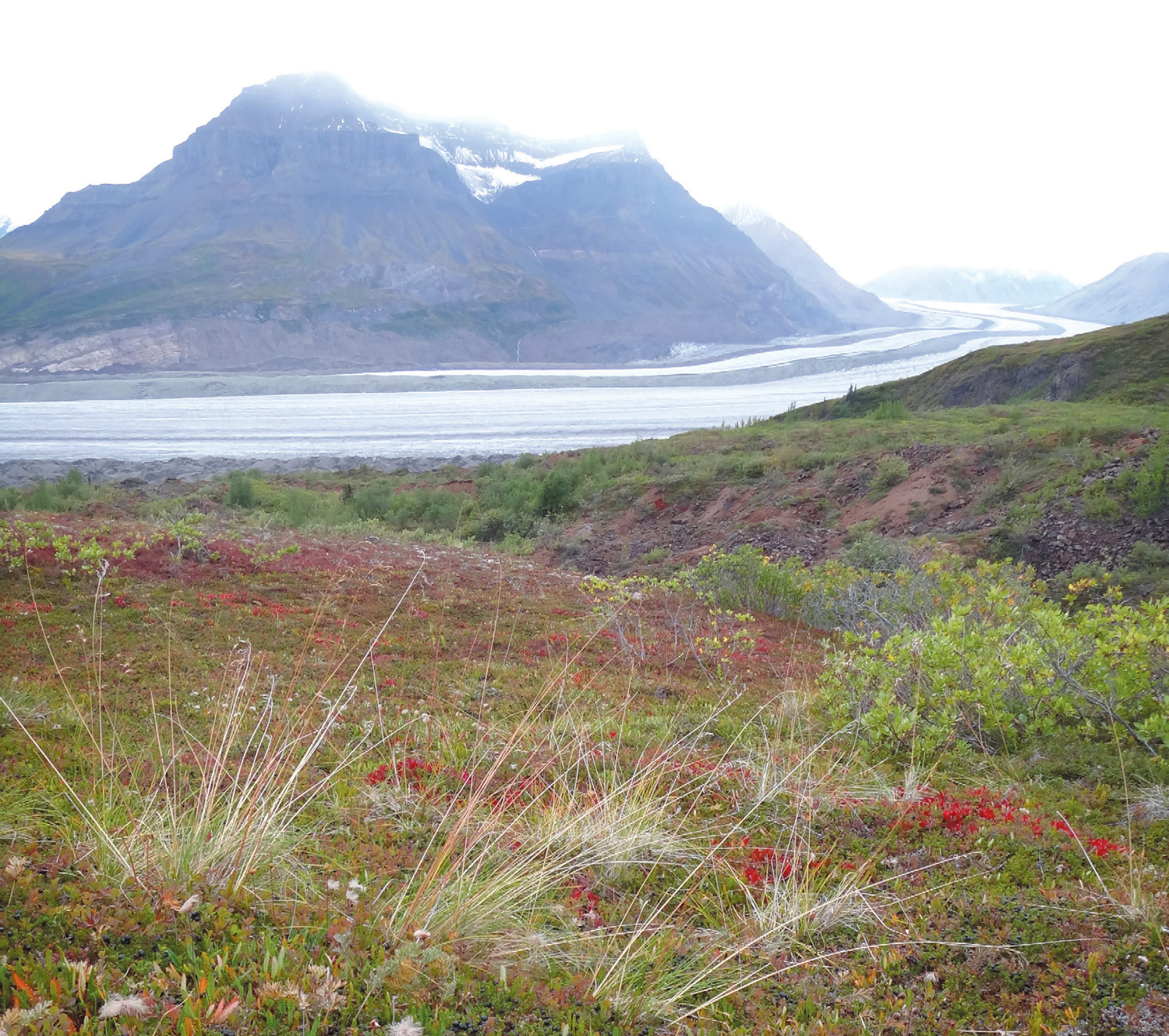A hazy outdoor landscape photograph captures a picturesque scene featuring a majestic, snow-capped mountain with two prominent peaks and steep slopes in the distance. The snow forms a bowl-shaped accumulation at the mountain's summit. Below, a river meanders from the left to the right side of the image, flowing in front of the mountain and snaking through the terrain. The foreground is characterized by rough, hilly terrain adorned with verdant, low-to-the-ground vegetation, including green moss-like plants and tufts of tall grass. Scattered throughout this colorful grassy field are small flowers of various hues, such as reds, yellows, and whites, adding a vibrant touch to the scenery. Some white weeds also sprout throughout the area, along with identifiable plants like broom weed and little red and orange flowers closer to the camera. The photograph's sky is an overexposed white, casting a hazy, almost blurred effect over the mountain peaks and diminishing the clarity of their details. This image is seemingly taken from an elevated, hilly vantage point leading down to the river, providing a detailed and layered view of the natural landscape.